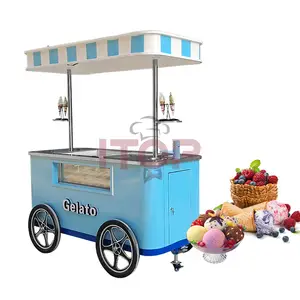This image captures a whimsical gelato cart, predominantly hued in powder blue, stationed centrally and slightly slanted from left to right. The cart's blue base is adorned with a small window displaying a variety of gelato flavors, and beneath this window sits a white sign with a black border simply inscribed "gelato." This charming structure is supported by two metal poles that hoist a tent-like roof, decorated with alternating blue and white blocks. To each side of the poles are two black spoked wheels, reminiscent of a sheriff's star. To the right of the cart, there are vibrant bowls of gelato in pink, yellow, and dark red, alongside a wicker basket brimming with fresh red strawberries. Within the setup, there's also a small, intricately colored pillow-like object in shades of orange, silver, and red, adding more texture and intrigue to the scene. The overall aesthetic, mixed with the bright assortment of colors like baby blue, white, red, pink, lemon yellow, and brown, evokes a joyful, inviting atmosphere, particularly appealing to children who might eagerly rush towards the gelato stand.